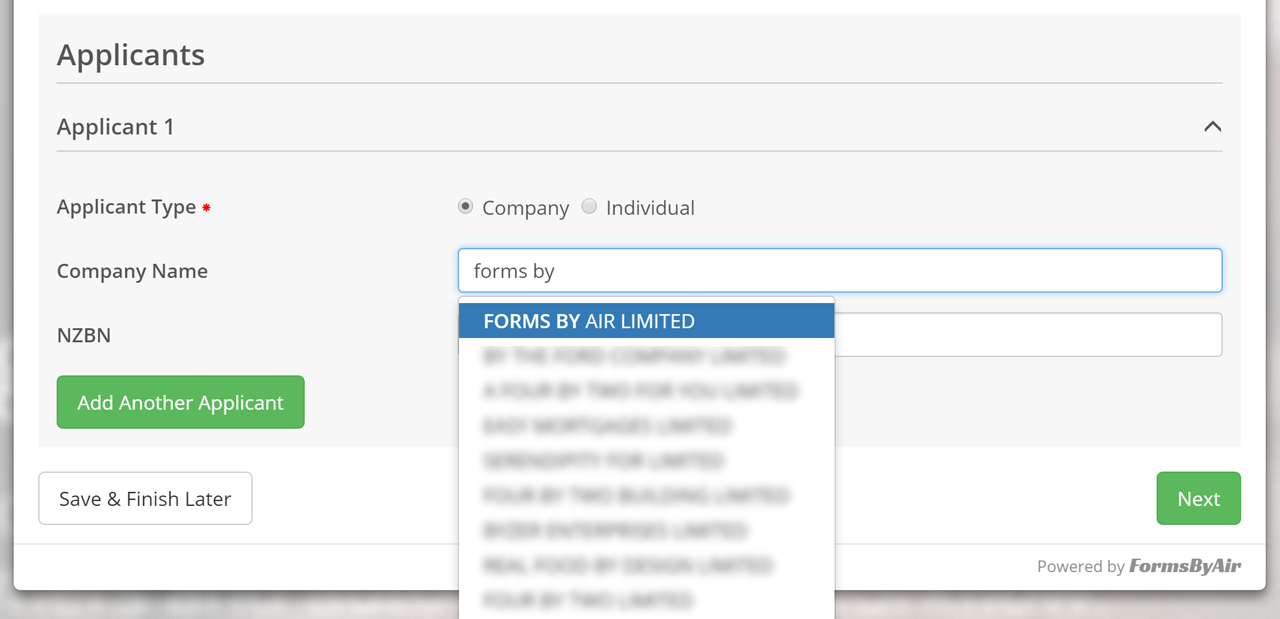Screenshot from an unidentified website showcasing an application form interface. The majority of the text appears in black against a white background. The header reads "Applicants" followed by the fields "Applicant 1" and "Applicant Type." A small red circle is positioned next to the word "Type."

Under the "Applicant Type" section, two radio buttons are available: one for "Company," which is selected, and another for "Individual." There is also a "Company Name" field, pre-filled with the term "Forms." 

A dropdown menu follows, with the first option displaying "Forms by Air Limited." This option is highlighted in a blue rectangle, featuring white uppercase text. Several lines below this selection are blurred out. 

The acronym "NZBN" is visible, accompanied by a search field partially obscured by the dropdown menu. 

Towards the bottom, a green rectangle button labeled "Add Another Applicant" in white text is present. To its left, a white rectangle button reads "Save and Finish Later." On the bottom right, a green square button marked "Next" in white letters is located. 

The footer of the interface notes "Powered by Forms by Air," with the text "FORMSBYAIR" capitalized and concatenated into a single string.